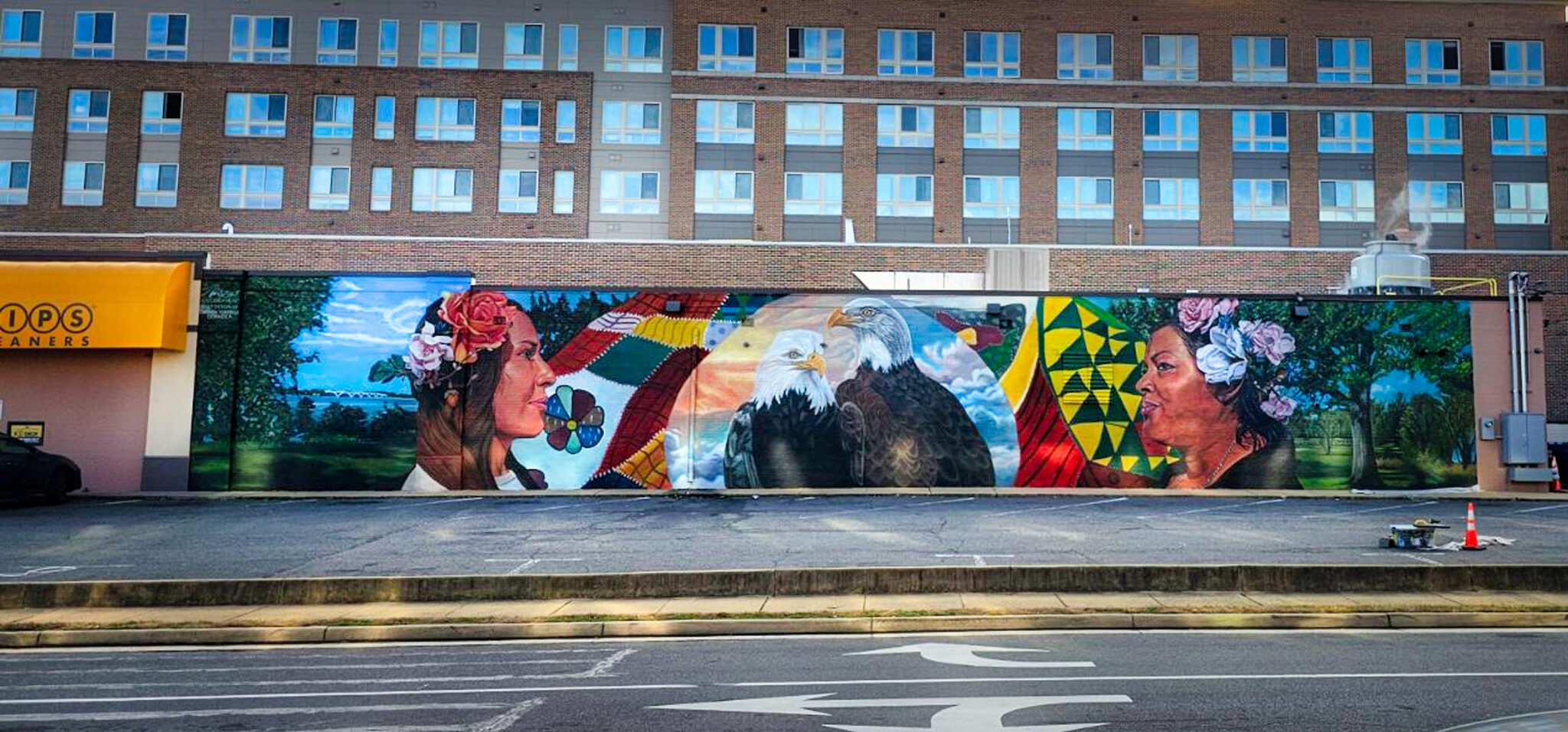A vibrant mural spans the entire length of a brick wall outside a building, blending the bold spontaneity of graffiti with the deliberate artistry of commissioned work. The wall stretches from left to right, completely covered in a cohesive and expansive piece rather than sporadic patches typical of traditional graffiti. The artwork features majestic bald eagles soaring amidst a surreal landscape where women emerge gracefully from blooming flowers. The vivid colors and intricate details suggest a professional touch, hinting that this may indeed be a commissioned masterpiece rather than an impromptu street art endeavor.